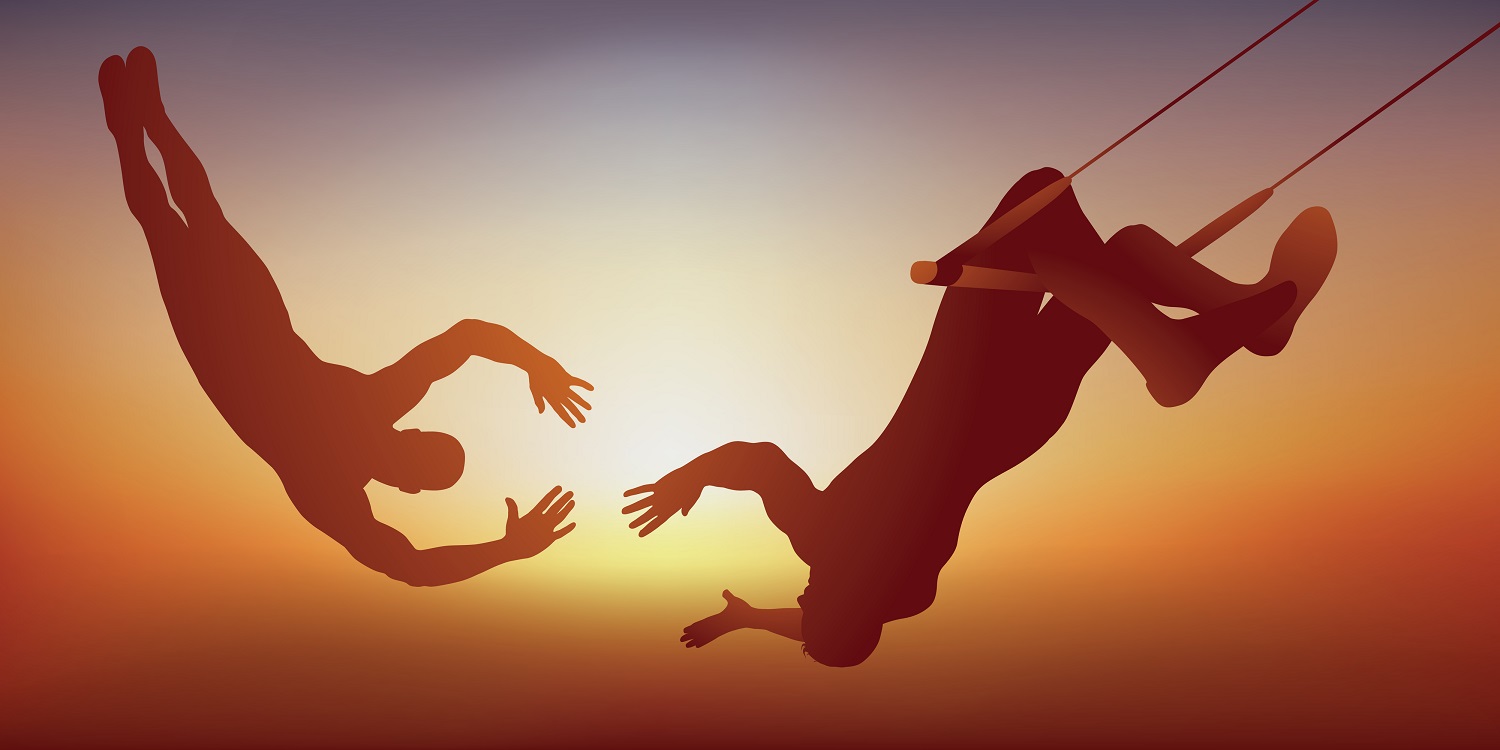In this AI-generated or digitally-drawn image, two trapeze artists are depicted in mid-air against a backdrop that transitions from deep to soft shades of amber, orange, yellow, white, and then gray, reminiscent of a sunset. One artist, upside down with pointed toes, is free-falling with outstretched hands, ready to grasp the other artist, who is hanging by his knees from a trapeze. The entire scene is rendered in a cartoon-style silhouette, emphasizing the dramatic, glowing haze behind the performers. The trapeze swing's ropes extend into the upper right corner of the image, enhancing the sense of suspense and motion as the two figures reach out to one another. The indistinct background leaves it ambiguous whether the scene is set in a circus tent or an open sky.